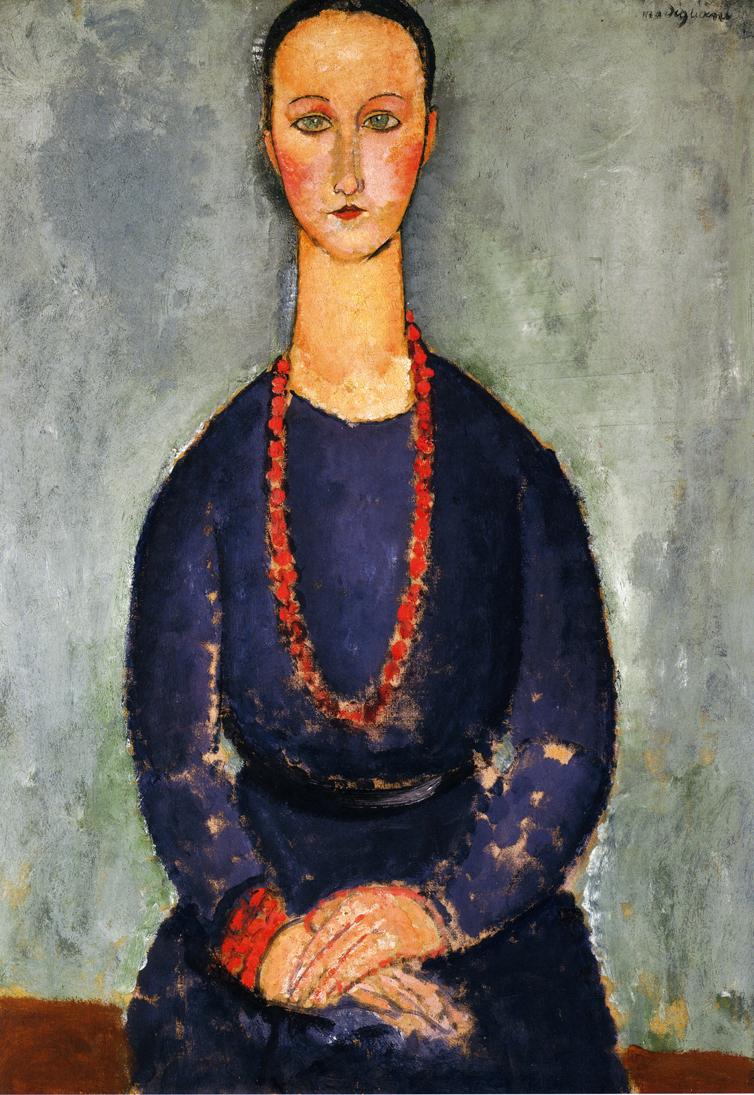The painting depicts a white woman posed against a predominantly faded blue-grey background. She has black hair styled into a very short cut or skullcap, revealing a slightly receding hairline, and her uniquely long neck adds an elegant, elongated appearance to her figure. Her facial features include close-set blue or green eyes, fine eyebrows, a long nose, rosy cheeks, and red lipstick. The woman is attired in a blue long-sleeve dress, which appears to be tattered and worn, and she accessorizes with red jewelry—a necklace and bracelets on her right arm. She sits with her hands folded demurely on her lap, possibly on a chair or bench, the details of which are partially obscured but visible as a brown section at the base of the image. An air of vintage artistry pervades the painting, suggesting it was created many years ago, and in the upper-right corner, faint, indecipherable letters hint at the artist's signature. The woman gazes directly at the viewer, her pose serene and contemplative.